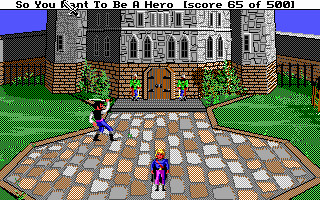This screen capture features a scene from a 1980s adventure computer game, reminiscent of the King's Quest series popular on Commodore and PC. The game's interface, wider than it is tall, showcases its era-typical primitive graphics with a limited color palette, likely either 4 or 16 colors. At the top of the screen, in gothic-style text, the game title "So You Want To Be A Hero" is displayed, followed by a score indicator showing "Score: 65 out of 500."

The scene itself presents a medieval castle with two guards flanking the gate, decked out in traditional guard attire. To the left of the guards stands a man dressed in pirate-like garb, wielding a sword raised over his right shoulder, with his back facing the viewer. Dominating the foreground is the game's protagonist, positioned at the center bottom of the image, standing on a large, stop sign-shaped cobblestone platform. This character is distinguishable by their blonde hair, blue cape, and pink pants, embodying the classic hero archetype of the era. The image captures a nostalgic moment from a golden age in computer gaming history.